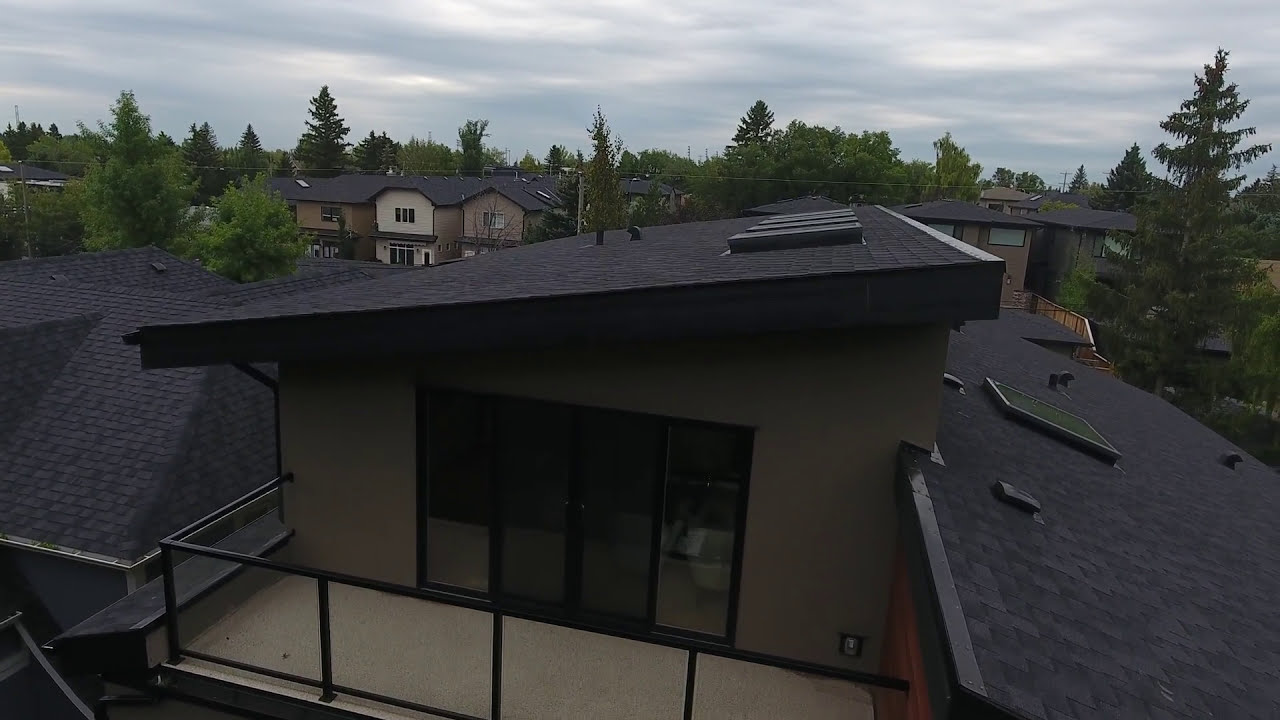The photograph, taken outside on a cloudy day, captures the top level of a house with detailed clarity. The main structure features a slightly raised left-hand side which showcases its dark beige exterior adorned with a set of glass sliding doors that lead out to a balcony. The balcony is secured with a dark grey metal handrail, providing a stark contrast against the facade. The black-tiled roof of the house is slanted, showing off a series of skylights—both square and protruding. Notably, there seem to be four skylights aligned along the top of the roof. The roof angles downwards, with one part slanting to the left and another part to the right.

To the right of this main structure, part of a grey slab roof with an additional skylight is visible, hinting at an adjacent structure or extension. In the top left of the composition, another house can be seen, sporting similar grey tiles and interspersed with tall trees. These trees, of varying heights, weave between several other houses visible in the background. Each of these buildings shares a common color palette of beige and light brown with dark-colored roofs, seamlessly integrating into the verdant, tree-filled landscape. The presence of multiple roofs and buildings in the background creates a layered, textured effect that emphasizes the interconnectedness of this residential area.